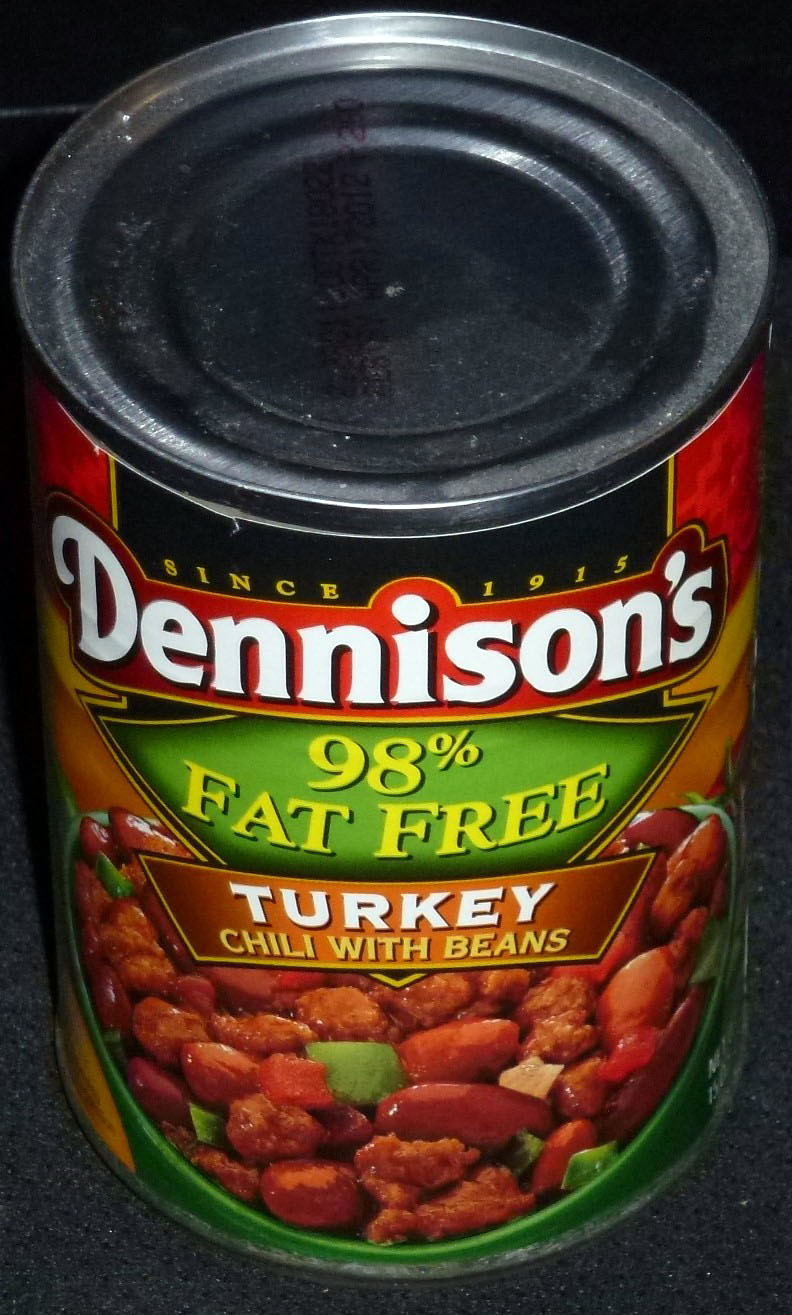The image features a can of Denison's Turkey Chili with Beans. The can's label showcases a vibrant red background with the brand name "Denison's" prominently displayed in white font. A section of the label highlights that the chili is "98% Fat Free" in green and yellow text. Further down, in a dynamic mix of green, yellow, and orange hues, the label identifies the product as "Turkey Chili with Beans."

A photograph of the chili is displayed on the label, offering a tempting preview of the contents. Visible are hearty chunks of brown turkey meat interspersed with red kidney beans. The dish also contains small green squares, possibly peppers, adding a subtle touch of color and texture. The chili is presented in a green dish, enhancing the visual appeal. The can is shown from an angled top view, allowing a glimpse of its silver lid.